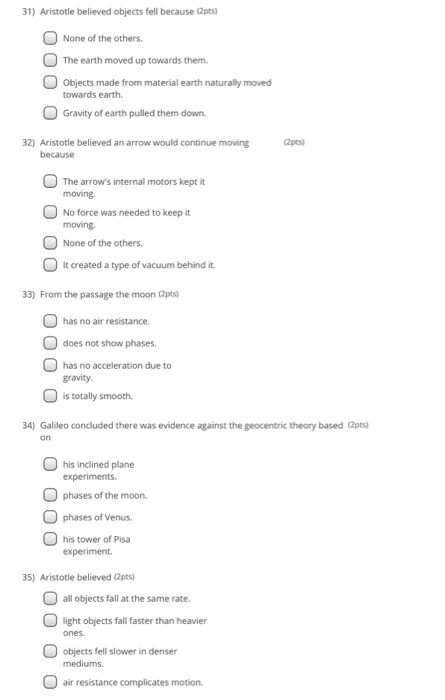This is a rectangular screenshot captured from a smartphone, showcasing an academic test or study material, likely for an examination. The background is white, providing a clean contrast for the primarily dark gray text. The image contains a series of questions, specifically numbered from 31 to 35, indicating this is part of a larger set of questions.

The questions cover topics related to historical figures such as Aristotle and Galileo, suggesting the subject matter is likely focused on science or philosophy. Each question is presented in a multiple-choice format, with empty checkboxes positioned to the left, ready for the test-taker to select their answers. Each question is worth two points, as indicated by the "(2PTS)" notation following each query.

Among the listed questions, question number 33 specifically refers to content from a passage titled "The Moon," and is accompanied by four answer choices. The text is relatively small, implying that a considerable number of questions have been compactly arranged within this single screenshot. The overall layout suggests an organized and structured approach to academic assessment.